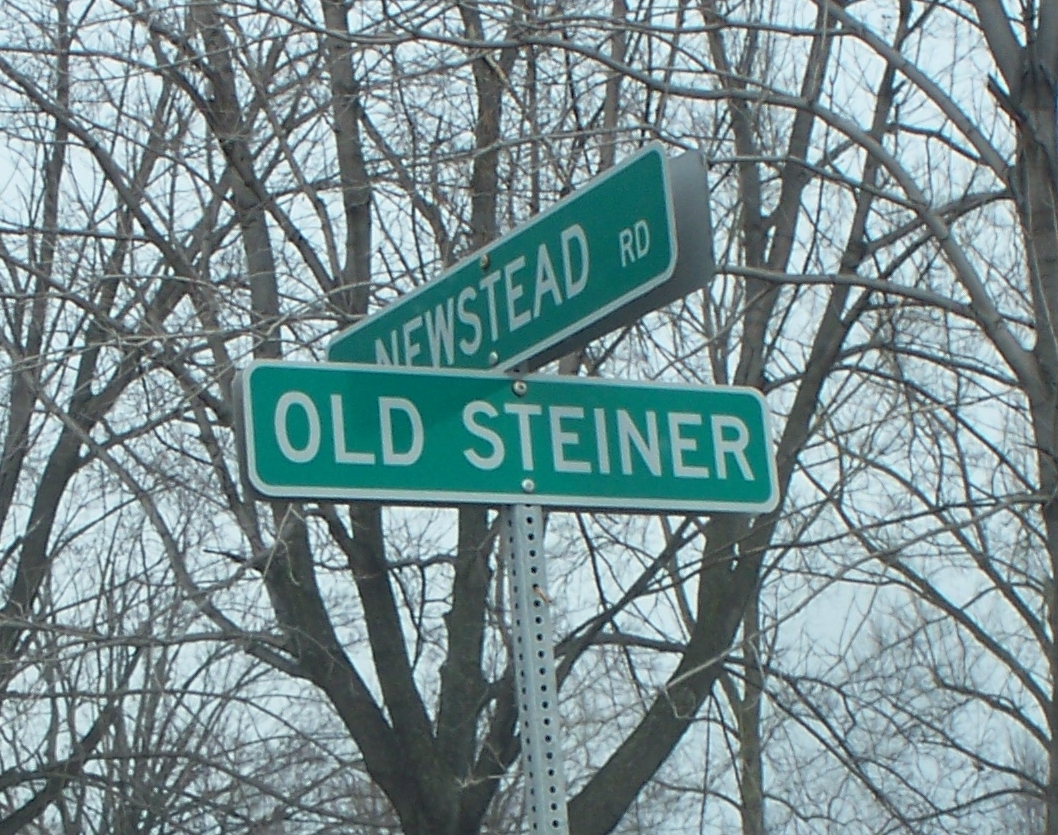A rectangular photograph depicts two street signs attached to a silver-colored, perforated metal pole that extends from the bottom of the frame. Centrally positioned, the pole supports a rectangular green street-name sign with a white border, secured by two bolts. The sign prominently displays "OLD STEINER" in large white capital letters. Above this sign, another street-name sign is affixed, oriented to the left rather than forward. This additional sign reads "NEWSTEAD R.D." in the same white capital text on a green background, also attached with two bolts. In the background, a cluster of trees, bare of leaves, fills the scene, providing a stark contrast to the signs in the foreground.